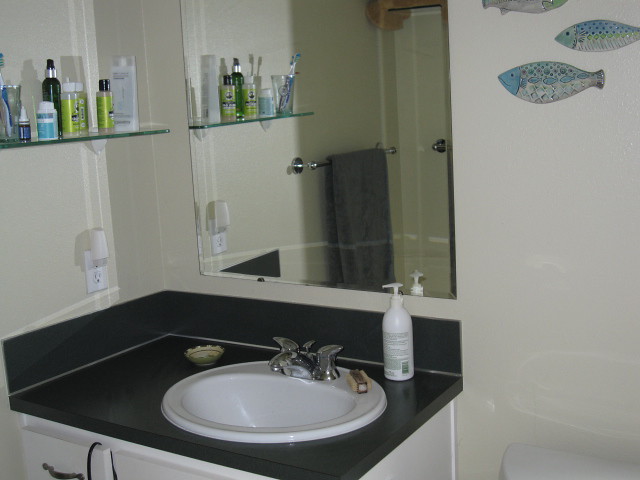The image depicts a meticulously organized bathroom. On the right side, a sleek glass shelf holds a variety of toiletries, predominantly green and white, with one blue and white item and another dark blue and white object. An electrical outlet is present, with an unidentifiable white object plugged into the top socket. This entire setup is mirrored on the right, extending the view to include two toothbrushes, a hanging towel, and part of a door. Below the glass shelf is a counter with a contrasting black surface and a white sink. On the counter sits a white pump bottle with green writing, a bar of soap on the sink, and a small green bowl. The lower left corner reveals a drawer with a black item draped over it, adding to the bathroom’s well-kept appearance.